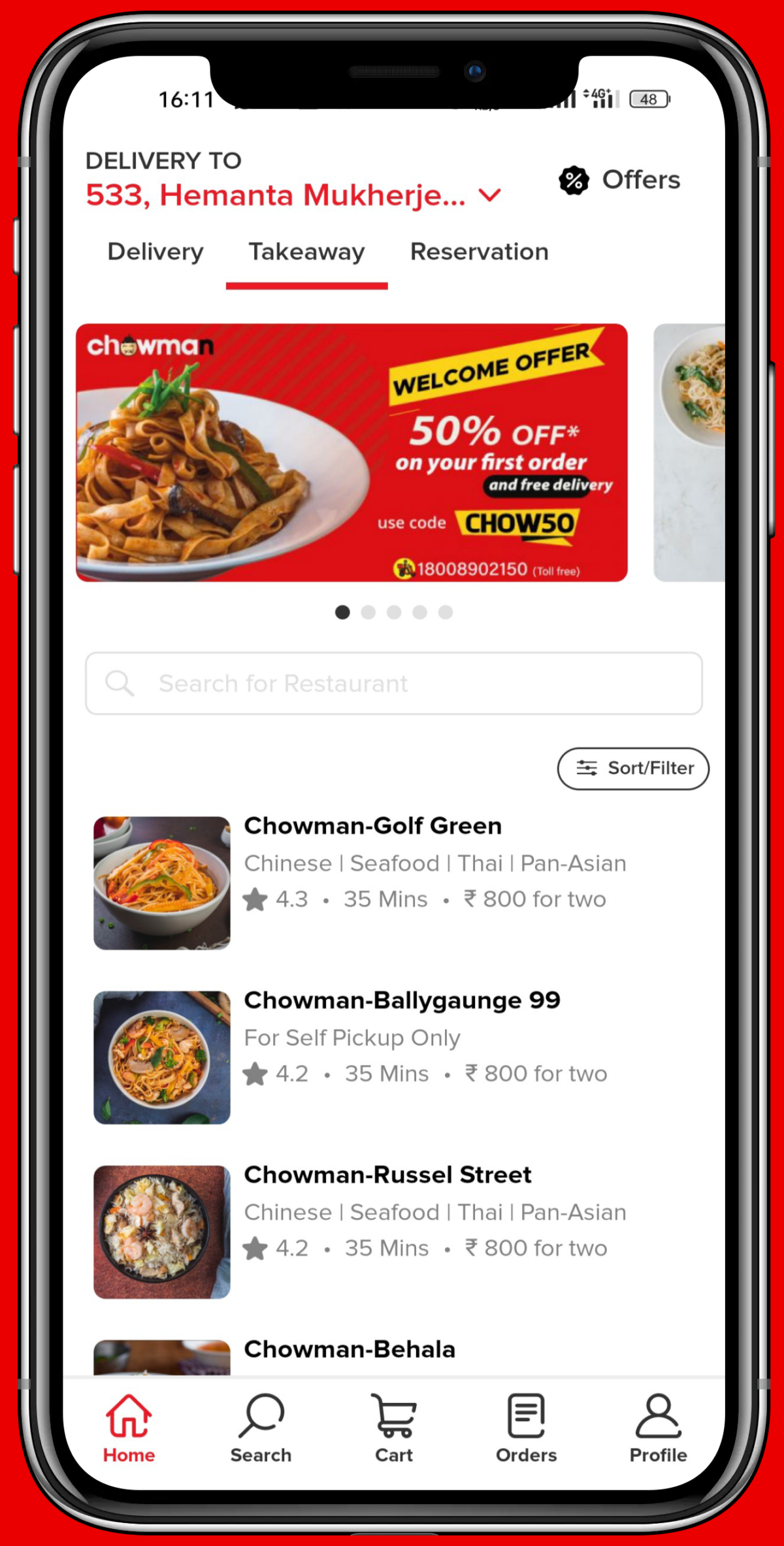In this vibrant advertisement image, a smartphone is prominently displayed, showcasing its sleek front profile. The power button is visible on the right side, while the left side features the notification switch along with the volume up and volume down buttons. The phone's screen is open to a food delivery service app.

At the top of the screen, there's a delivery address field indicating "Delivery to 533 Himanta, Mukherjee." Adjacent to it on the right is an "Offers" button. Below this section, there are three main options: "Delivery," "Takeaway," and "Reservation," with "Takeaway" being selected.

The next section prominently features a Truman advertisement announcing, "Welcome Offer: 50% off on your first order and free delivery." The promo code is "CHOW50." Following this is a search bar prompting users to "Search for restaurants."

The list of restaurants displayed includes:
1. Chow Man, Golf Green
2. Chow Man, Bally Gang 99
3. Chow Man, Russell Street
4. Chow Man, Bahala

At the bottom of the screen, there is a navigation bar with five buttons, each accompanied by corresponding symbols. These buttons are labeled "Home," "Search," "Cart," "Orders," and "Profile."